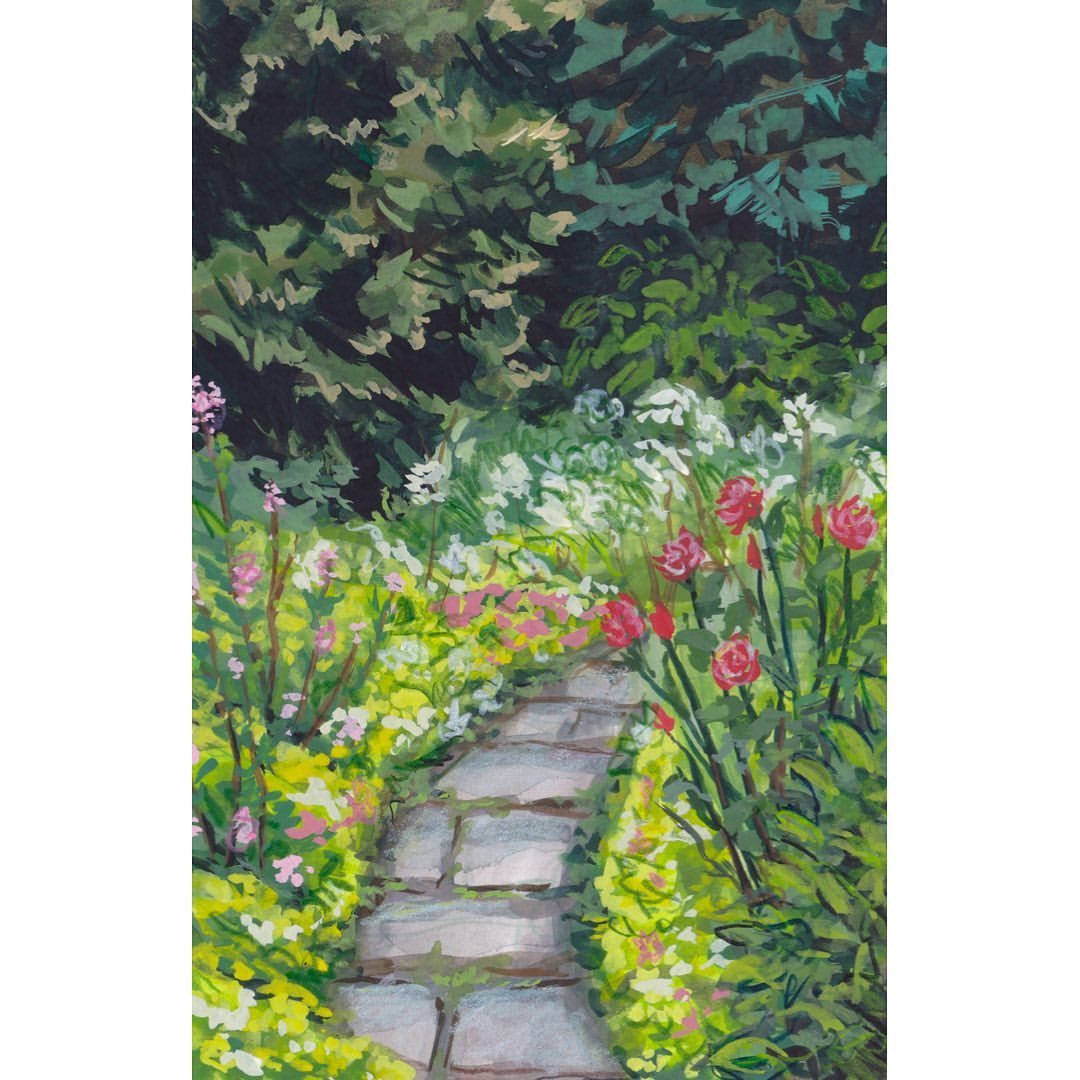This painting, rendered in an Impressionistic style with smudged, blurred details, depicts a meandering cobblestone pathway that begins at the center and curves gently to the right, disappearing into the dense greenery. The pathway is composed of square stones set into the soil, and it winds through a lush garden area before vanishing into a woodland of tall, dark greenery and notably indistinguishable tree trunks. 

On both sides of the pathway, vibrant flora flourishes in a cacophony of colors. To the right, the garden features clusters of red and maroon roses with their long stems prominently rising above the ground cover, interspersed with additional white and pink flowers. There are also possible yellow flowers, perhaps daffodils, adding to the vivid display.

To the left, the garden bursts with taller white flowers and prominent large purple blossoms, possibly lilacs, standing against a backdrop of smaller pinkish flowers. Further contributing to the garden’s rich tapestry are yellow and pink flowers, which might include orchids, rising among the dense vegetation.

The upper portion of the painting is dominated by a canopy of thick foliage, contributing to a sense of enclosure and making the sky completely invisible. This foliage consists predominantly of leafy greenery, suggesting an encompassing forested area. The overall composition evokes a serene, almost mystical garden pathway leading into a verdant, tree-shrouded retreat.